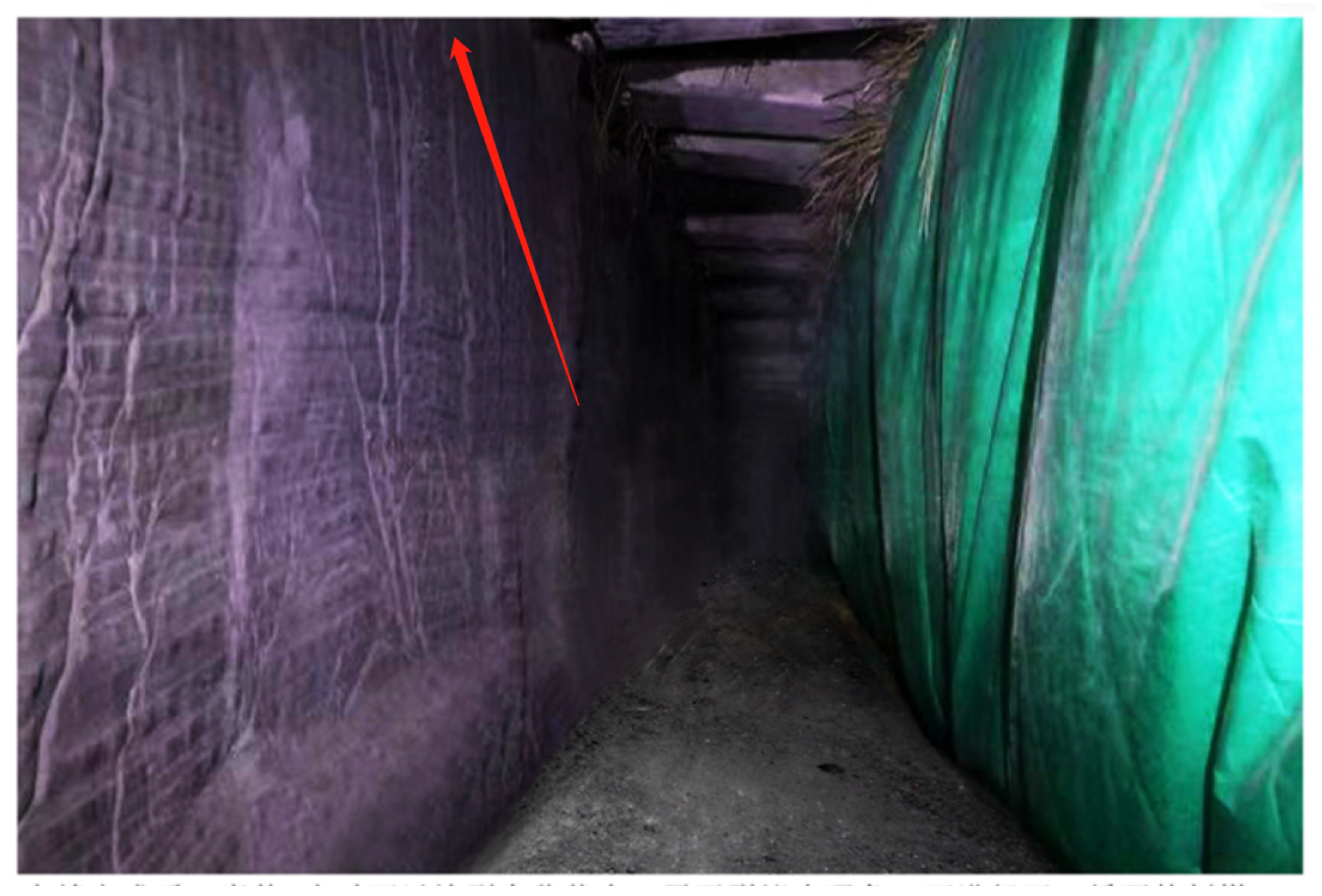The photograph depicts a narrow, indoor or potentially underground tunnel with a rectangular shape measuring approximately five inches wide by four inches high. The floor of the tunnel appears to be a gray cement pathway, starting from the bottom center and narrowing to a point as it extends into the distance. The left-hand wall, which is sheer or carved from stone, features numerous horizontal striations and indentations with a purplish tone. The ceiling of the tunnel stretches across the entire width at the top of the image and consists of horizontal wooden beams with bits of straw protruding from them. A long, thin red arrow originates near the center of the image, pointing upward but not revealing its destination.

On the left side of the image, the stone wall's texture adds a rugged aspect, while on the right side, a green tarp hangs from the ceiling to the floor, possibly concealing something behind it. Scattered bits of grass or hay are visible on both the floor and the straw-covered beam area, adding an organic element to the scene. Despite the low lighting and possible blur, these distinct features give the tunnel an eerie and mysterious atmosphere.